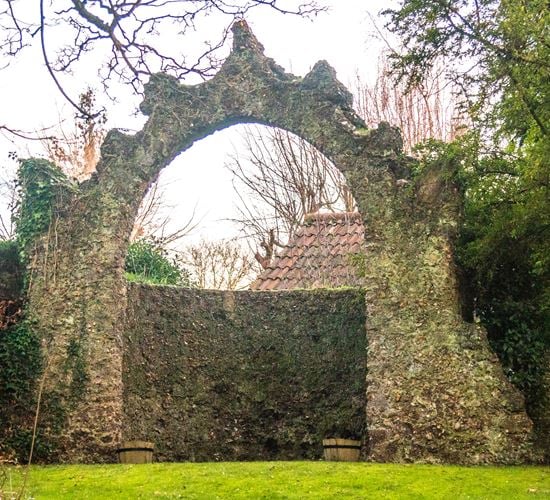The photograph captures an outdoor garden scene dominated by an ancient stone arch, weathered and covered in moss, stringy branches, and leaves. The arch, which has a crown-like top, frames a stone alcove that is partially obscured by the erosion of time. At the base of the arch are two half-barrel wooden planters, each with a black rim. The surrounding area is lush with bright yellow-green grass and an array of trees, some evergreen and others barren. In the background, a stone wall that appears brittle and deteriorated can be seen along with the roof tiles of a house, partially concealed by the architecture. Above, the sky is gloomy and cloudy, while stray branches encroach from the top of the frame, adding to the intricate detail and historical ambiance of the scene.